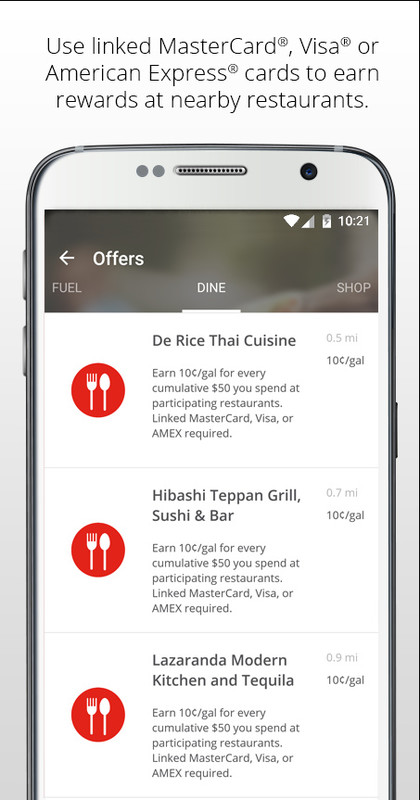In this image, we see an advertisement encouraging the use of linked MasterCard, Visa, or American Express cards to earn rewards at nearby restaurants. The advertisement prominently features a smartphone screenshot with an app interface. At the top center, the text reads: "Use linked MasterCard, Visa, or American Express cards to earn rewards at nearby restaurants."

In the upper left corner of the app, there are four tabs labeled "Offers," "Fuel," "Dine," and "Shop," with the "Dine" tab selected. Below, three restaurants are listed with details. The first restaurant is "Day Rice Thai Cuisine," the second is "Hibachi Teppan Grill Sushi and Bar," and the third is "Lazzaranda Modern Kitchen and Tequila." Each restaurant listing includes a description: "Earn 10¢/gal for every cumulative $50 you spend at participating restaurants. Linked MasterCard, Visa, or Amex required." Additionally, the distance to each restaurant is displayed on the right side of the screen.

On the left side of each listing is a consistent symbol: a red circle containing a white fork and spoon.